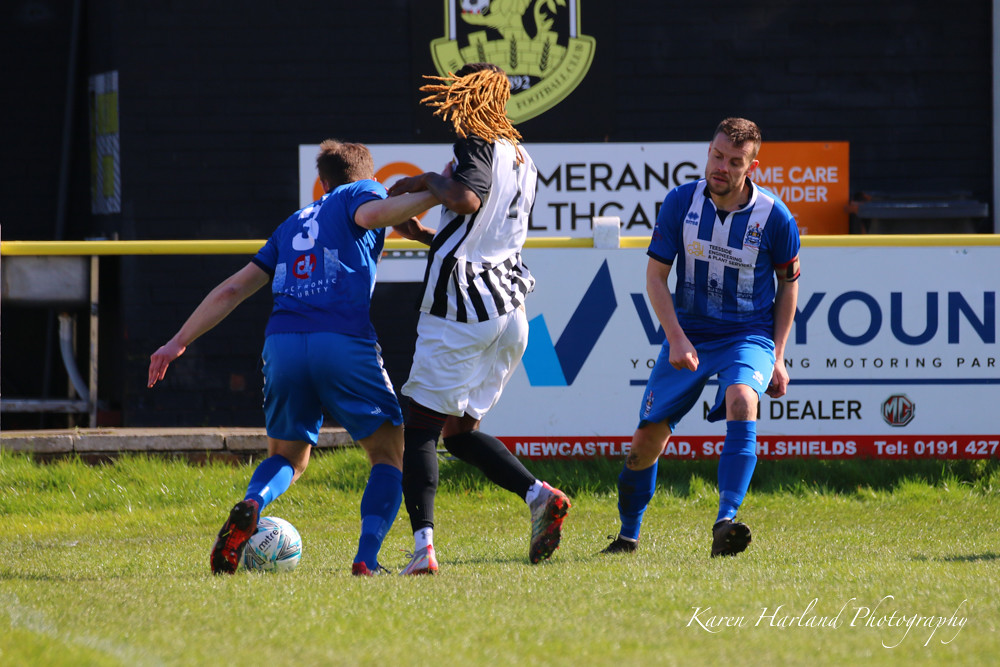The image captures a lively moment in a daytime outdoor soccer match on a lush green field. Central to the scene are three players engaged in a dynamic play. On the left, a player in a blue and white uniform, identified by the number three on his jersey, is about to kick the ball positioned near his left foot. To his immediate right, an opposing player with light brown dreadlocks, dressed in a black and white striped uniform, attempts to block the kick by intertwining his arm with number three's. Another player in a blue and white uniform stands further to the right, slightly facing the camera. In the background, various advertisements and fixtures, including a low stone wall, a yellow fence bar, and signs for a motoring dealer and a home care provider, provide context to the location. A barely visible football club logo featuring a lion can be seen among the background elements. At the bottom of the image, the signature "Karen Harland Photography" is elegantly scripted in white letters on the green grass.